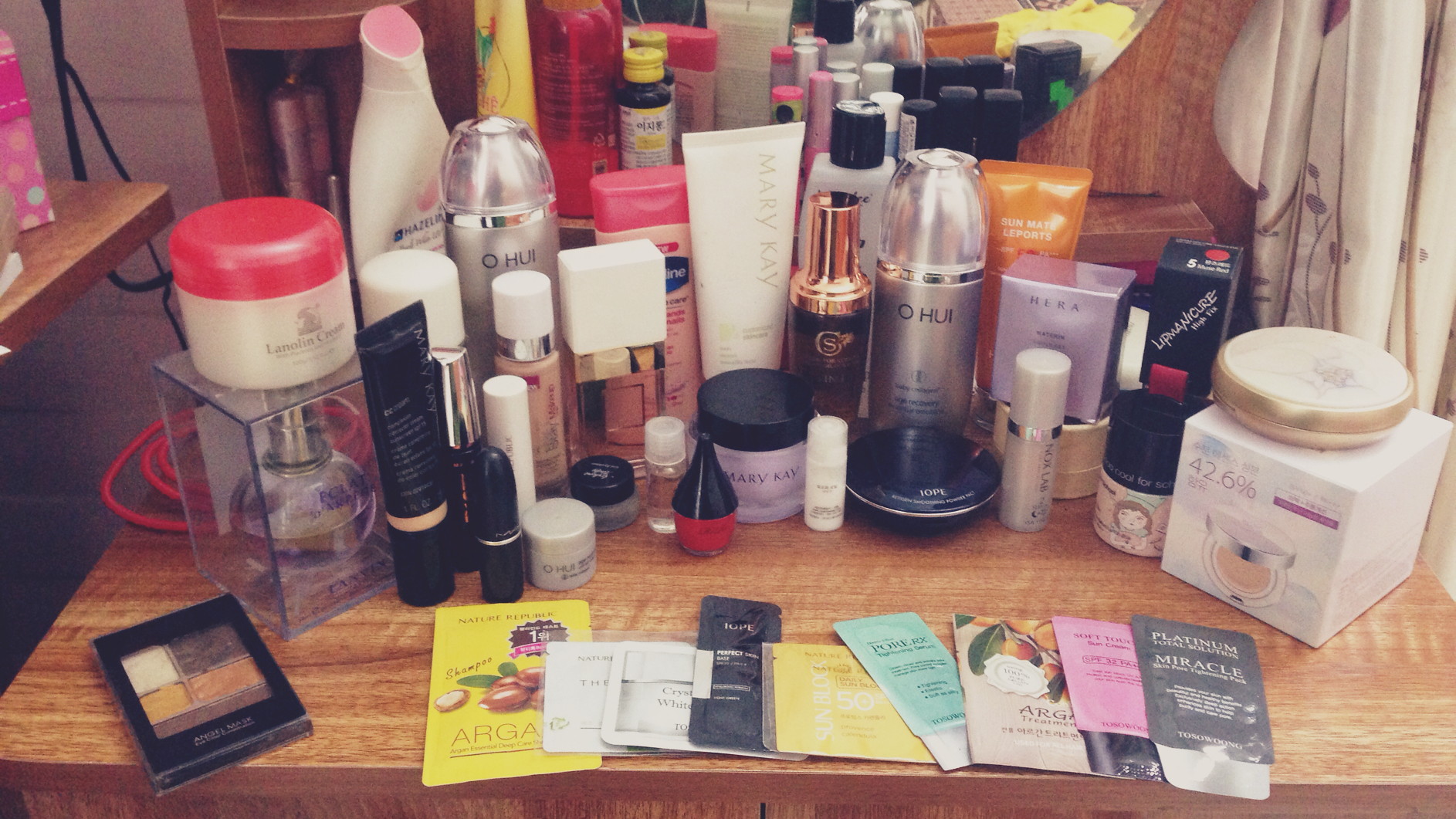On a brown table, a diverse collection of beauty products is meticulously arranged. A small glass container hosts a delicate bottle of perfume, topped by a white container with a striking red lid. Below this, to the left, lies a compact eyeshadow palette. To the right of the glass container, a sleek black bottle, likely foundation, stands beside a taller silver bottle and a white bottle with a pink lid. Moving towards the center, a white lotion bottle emblazoned with the Mary Kay logo takes prominence, flanked by yet another tall silver bottle. Additional bottles include a distinctive purple perfume bottle, whose counterparts are reflected in the mirror behind them. On the far right, a white box features the image of a foundation jar. Nearby, several flat containers house samples, possibly of lotions or perfumes; one notable sample is yellow and labeled with "argan oil." The array concludes with a black flat container, anchoring the collection.